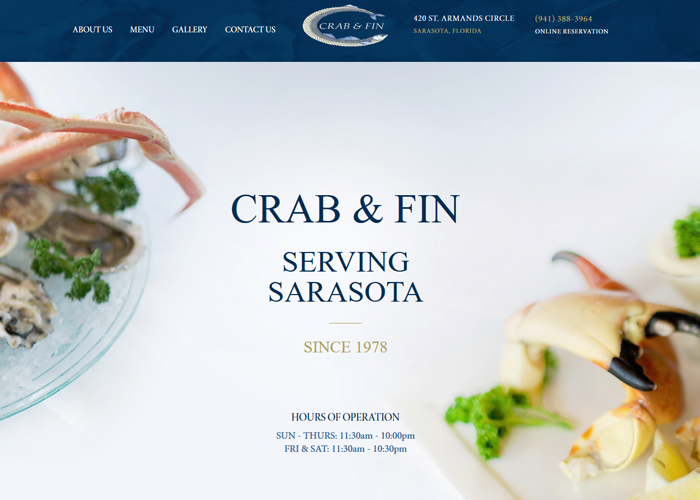**Detailed Caption:**

This image is a screenshot of a web page for a restaurant named "Crab & Fin." At the top of the page, there's a solid blue navigation bar. In white text on the left-hand side, it says "About Us," followed by "Menu," "Gallery," and "Contact Us" as you move towards the right. 

In the center of the blue bar, there is a logo featuring a fish inside a circle, with "Crab & Fin" written inside. To the right of the logo, the address "420 St. Armand's Circle" is displayed, followed by "Sarasota, Florida" in green text. Further right, the phone number "941-358-3964” is also in green. Beneath these details, "Online Reservation" is written.

Below the navigation bar, there's a main image. On the left-hand side of this image, there's a transparent plate showcasing three crab legs, a few oysters garnished with parsley, and some wedges of lemon. On the bottom right of the image, there's a small white bowl containing two black-tipped crab claws, also garnished with parsley and lemon wedges.

Centered between the image elements, "Crab & Fin" is written in dark blue text. Below this, "Serving Sarasota" is also in blue, followed by "Since 1978" in gray text. Further down, "Hours of Operation" is listed in blue, detailing the opening hours: "Sun-Thurs: 11:30 AM - 10:00 PM" and "Fri & Sat: 11:30 AM - 10:30 PM."